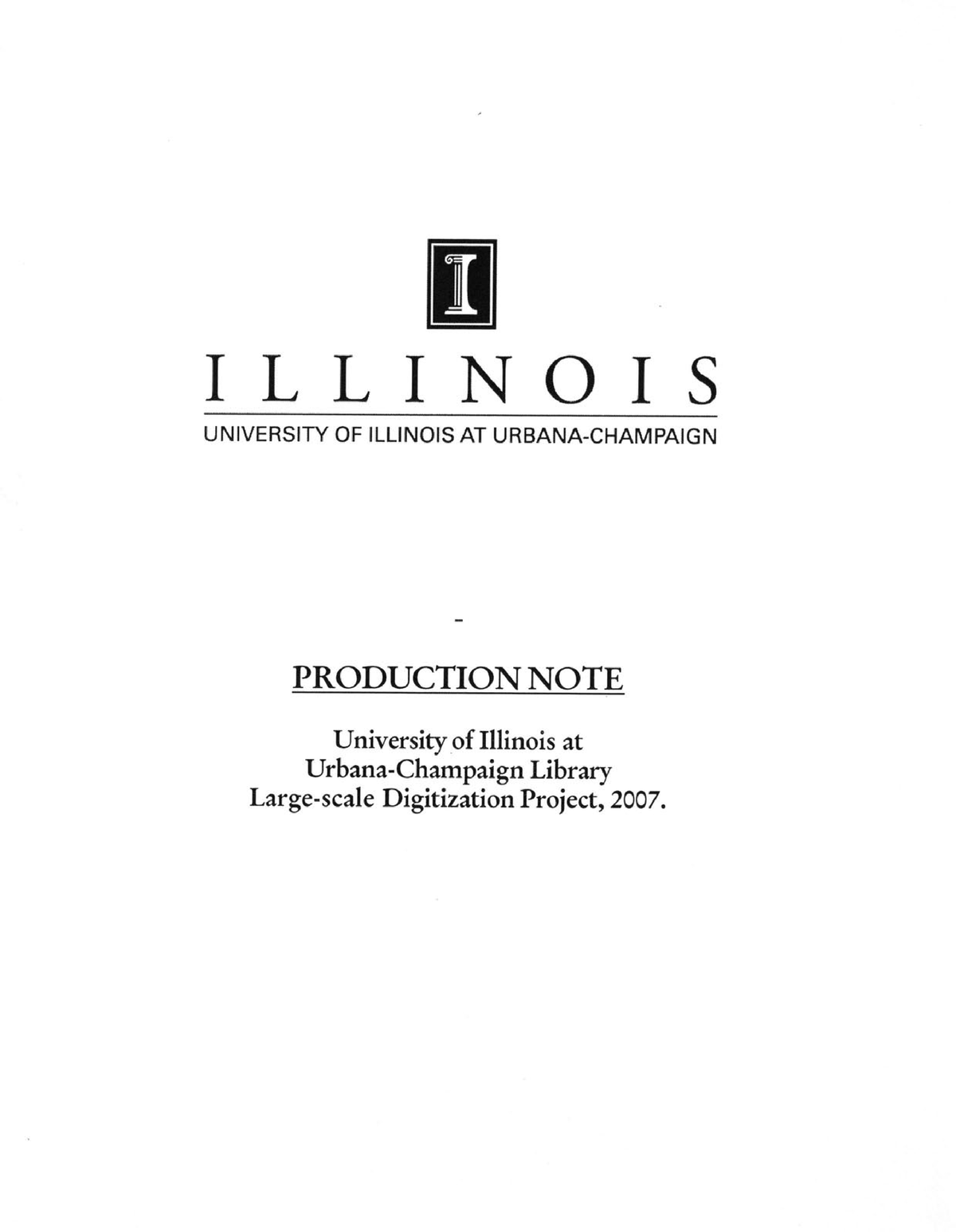This image appears to be the cover page for a document from the University of Illinois at Urbana-Champaign. The background is white, prominently featuring a black and white bordered square at the center. Inside the square, set against a black background, is a large white letter 'I' rendered in an etched and shaded font with black shading. Below this emblem, the word "Illinois" is centered in black lettering, followed by a horizontal black line.

Further down, centered text reads "University of Illinois at Urbana-Champaign." In the lower portion of the page, in a footnote-like area, there's a single dash, under which "Production Note" is displayed in large, bold black font, also underlined in black. Lastly, the address for the university is provided: "University of Illinois at Urbana-Champaign Library. Large Scale Digitization Project, 2007."